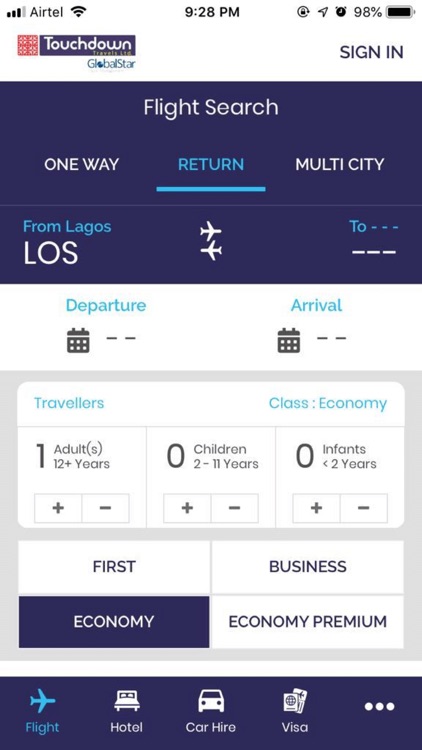The image depicts a smartphone screen displaying a flight search page for Touchdown Global Star. At the very top, the status bar shows the current time as 9:28 p.m., the networking service provider as Airtel, Wi-Fi connectivity, and battery life at 98%. Additional icons include an alarm clock, a send button, and another symbol that seems to be for lock, search, or reload.

The main header of the page reads "Touchdown Global Star," with an option to sign in on the right side, which indicates that no user is currently signed in. The primary section of the screen focuses on a flight search interface. Users can select between one-way, return, or multi-city flights, with the current selection being a return flight from Lagos (LOS airport). 

Below, users can input the departure and arrival dates, choose the number of travelers, and specify the travel class, which is set to economy. Options for travelers include adults, children, and infants, with categories of travel classes being economy, business, or economy premium. 

At the bottom of the screen, the flight search option is highlighted, with additional options like hotel booking, car hire, and visa services. There is also a three-dot menu that hints at more choices if clicked.